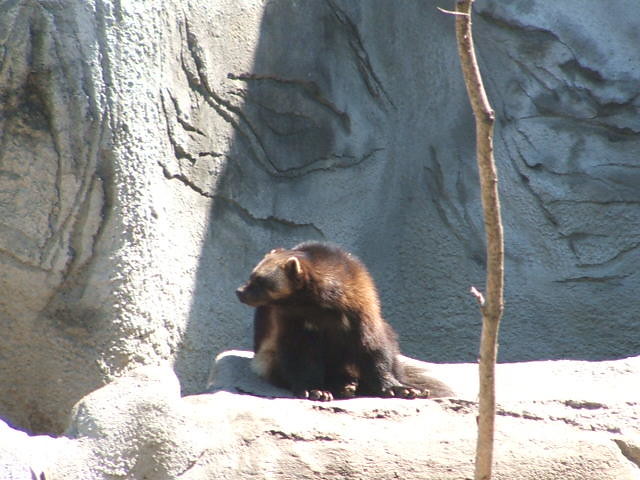Captured in a photograph outdoors during the daytime, this image depicts an older light brown wolverine, resting on what appears to be a replica plastic rock. The setting resembles a zoo enclosure, characterized by a rocky backdrop with sunlit and shadowed areas; notably, the sunshine highlights the wall while shadows obscure about half of the scene. The rock face in the background is grey from the mid-ground up and has intricate creases etched vertically on the left side and horizontally in the middle and right sections. In the foreground, a single, barren tree branch, devoid of leaves, adds a natural element to the composition. The wolverine, slightly hunched and emitting an aura of weariness, gazes downward and toward the left, revealing its predominantly dark brown fur with distinctive features: a white stripe running down its chest and white patches near its eyes and on the top of its head. Some of its fur also shows lighter, orangey tones, adding depth to its coat's coloration.